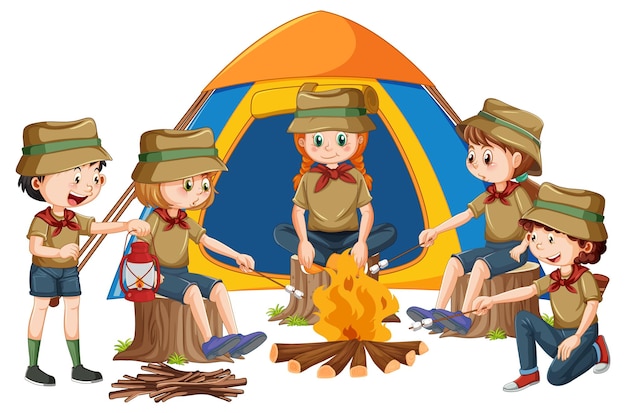The image is a detailed clipart illustration of five children, who appear to be campers, gathered around a campfire on a white background. Central to the image is the campfire, with three children seated on stumps and one child on the far right kneeling on one knee. The child on the far left is standing and holding a lantern. Each of the other four children is holding a marshmallow on a stick. Surrounding them are gathered sticks. 

The campers are uniformly dressed in blue pants or shorts, brown shirts with red scarves, and brown bucket hats featuring green stripes. Their footwear varies among blue, red, and green shoes. One camper is notably wearing green socks. The children have diverse hair colors, with most having dark brown hair, one child with blonde hair, and another with red hair.

Positioned behind the group is a multi-colored tent: its body is blue, the top is orange, and the opening is yellow. The visual is vibrant and high-quality, with no textual elements. The setting includes elements typical of a camping scene, but the absence of a detailed background underscores the clipart style of the illustration.